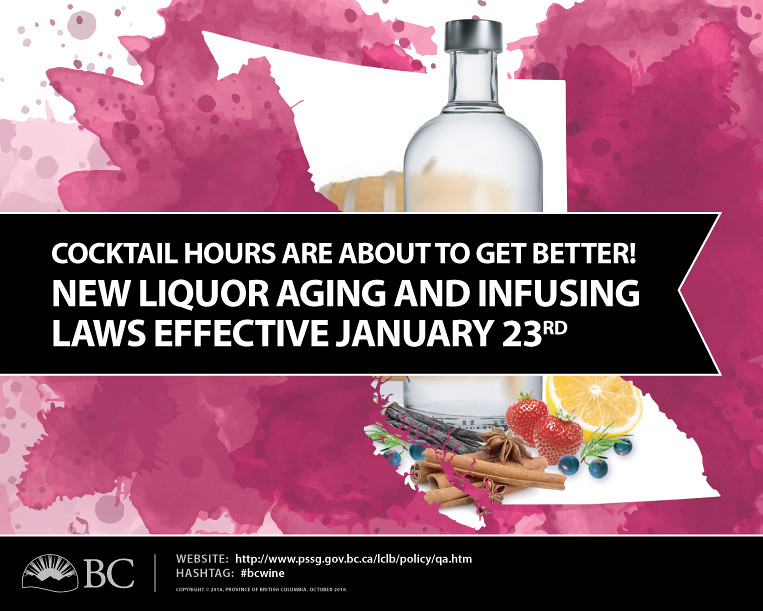This detailed promotional graphic serves as an announcement for new liquor aging and infusing laws effective January 23rd. The background is a striking magenta-colored watercolor splatter, resembling wine stains, set against a white canvas. Dominating the right third of the image is a clear, glass Absolute vodka bottle. Below and around this bottle, various ingredients are artistically arranged: a pile of cinnamon sticks with a star anise, two strawberries, an orange half, blueberries, vanilla beans, and rosemary sprigs. Overlaying the scenic backdrop is a black banner with three lines of prominent white text: "Cocktail hours are about to get better! New liquor aging and infusing laws. Effective January 23rd." At the bottom of the graphic, another black banner features smaller white text including a BC (British Columbia) logo on the left, accompanied by a website and a hashtag, providing additional resources and related social media information.